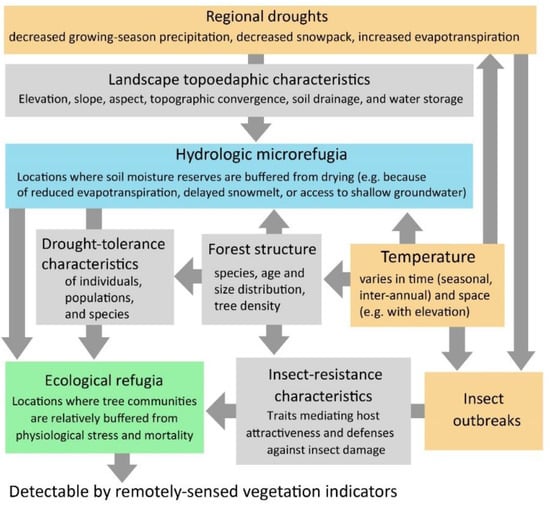The image is an intricate infographic or flowchart detailing factors impacting ecological micro-refugia. At the top is a light orange or beige rectangle that outlines key climate stressors: regional droughts, decreased growing season precipitation, decreased snowpack, and increased evapotranspiration, all presented in grey text. A grey arrow directs attention downward to the next level, labeled "landscape topographic characteristics," including elevation, slope, aspect, topographic convergence, soil drainage, and water storage.

Following that is a section labeled "hydrologic micro-refugia," explaining areas where soil moisture reserves are protected from drying due to factors like reduced evapotranspiration, delayed snowmelt, or access to shallow groundwater. This section is connected by multiple arrows to several other boxes. Below, the chart further subdivides into boxes titled "drought tolerance characteristics," "forest structure," and "temperature." From the "drought tolerance characteristics" box, an arrow leads to "ecological refugia." The "forest structure" box points towards "insect-resistant characteristics," while the "temperature" box leads to "insect outbreaks."

At the bottom of the "ecological refugia" box is a green box pointing to the use of "detectable by remotely sensed vegetation indicators." This chart integrates various interconnected factors to illustrate the complexity and resilience of hydrologic micro-refugia in ecosystems.